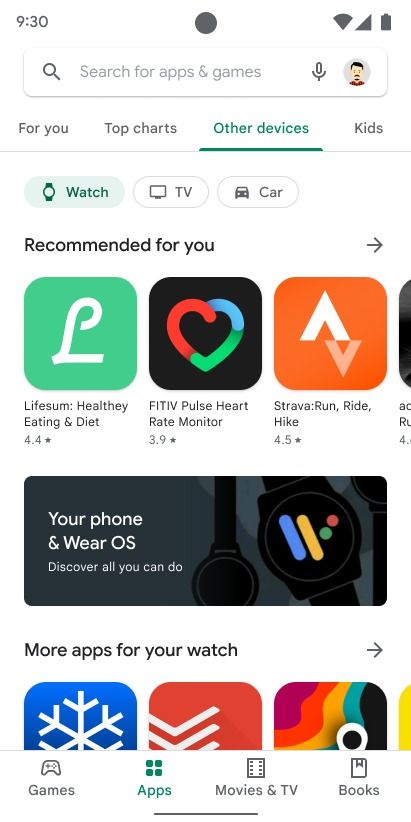The image appears to be a screenshot taken from a smartphone. The background is primarily white, and it displays what looks like an app store interface. Here's a detailed description of the screen:

- **Top Section**: The upper left corner shows the time, "9:30". Next to the time is a grayish-black circle, possibly indicating a notification or a service. On the right side of the top bar, a full battery icon is visible.

- **Search Bar**: Below the top bar is a search bar that reads “Search for apps & games”.

- **Category Tabs**: Under the search bar, there are categories to choose from: "For You", "Top Charts", "Other Devices", and "Kids". The "Other Devices" category is highlighted.

- **Subcategories**: Within "Other Devices", subcategories are presented: "Watch", "TV", and "Car". The "Watch" subcategory is selected and highlighted in green.

- **Section Headers and App Listings**:
  - **Recommended For You**: This section suggests three apps:
    1. **Lifesum**: Represented by a green icon with an 'L'. The full name is "Lifesum: Healthy Eating & Diet".
    2. **Fit IV Pulse Heart Rate Monitor**: Shown with a black circle icon featuring a heart colored in red, green, and blue.
    3. **Strava**: Displayed with an orange square icon. The full title is "Strava: Run, Ride, Hike".

  - **Your Phone & Wear OS**: This area features a gray rectangle with information likely about syncing or using Wear OS, titled "Discover All You Can Do".

  - **More Apps for Your Watch**: Highlights additional app recommendations with distinct icons:
    1. An app with a green icon and a snowflake.
    2. Another app with an orange icon featuring pointed lines.
    3. The final app has a multicolored icon with maroon, orange, yellow, teal, and black.

This screenshot appears to be part of an app store interface, specifically tailored to suggesting applications for a smartwatch.